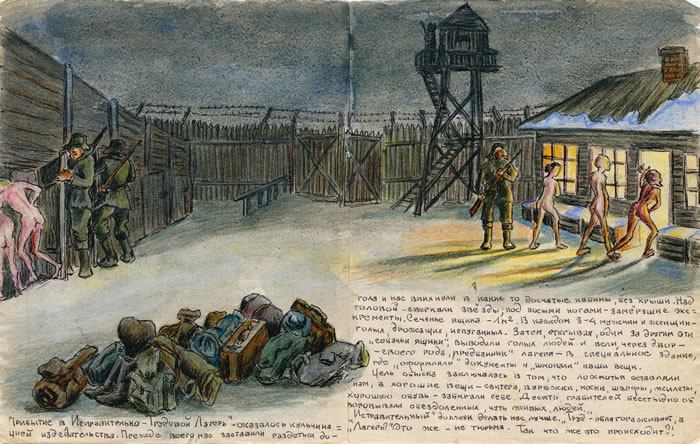The detailed, hand-drawn image vividly depicts a grim scene set in what appears to be a prisoner camp surrounded by a wooden fence topped with barbed wire and spikes. A tall wooden watchtower stands ominously in the background, complete with steps leading up to it. The ground is covered with snow, emphasizing the cold, harsh environment. The drawing features soldiers in warm uniforms with hats and boots, each holding rifles. On the right side of the image, a soldier stands guard as three naked individuals are being escorted into a building with a snow-covered roof and lights that hint at the bleakness inside. To the left, another pair of soldiers stand menacingly behind two naked men near a fence. The bottom left corner reveals a pile of the prisoners' belongings—bags, backpacks, helmets, and various sacks—suggesting they have been stripped of all personal items. The scene is rendered in muted colors, with browns, yellows, and whites from the snow dominating the palette. There is text in an unknown language located at the bottom right and left of the image, adding to the unsettling, mysterious nature of the scene. The clear, crisp detail of the drawing intensifies the sense of oppression and despair, making it an impactful visualization of a sorrowful moment.